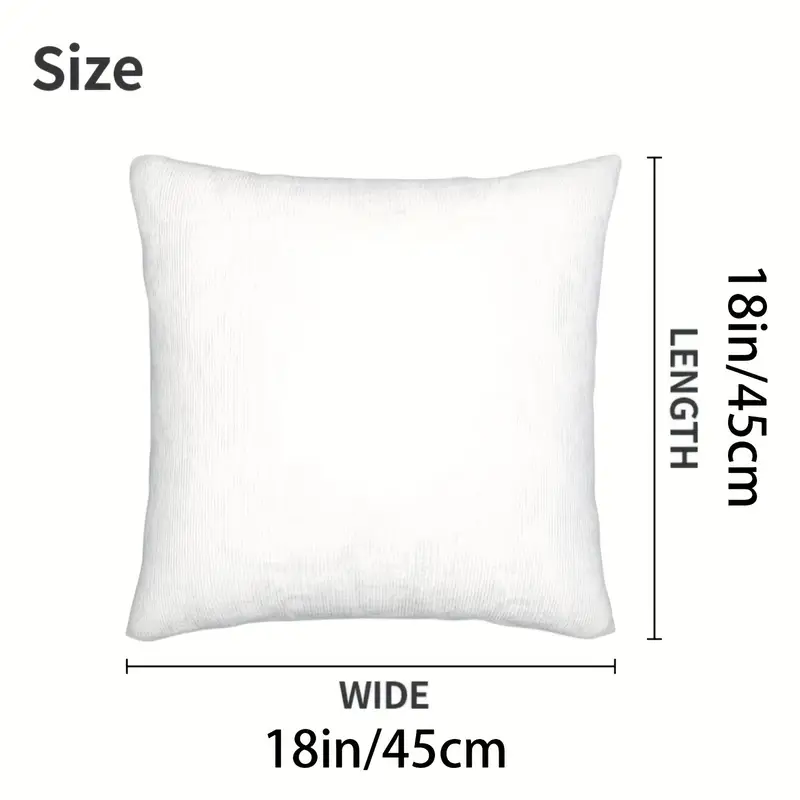The image is a detailed diagram of a plain, square white throw pillow against a white background. The text in the image provides specific measurements, indicating the pillow's size. In the upper left corner, there is black text that simply states "size." The dimensions of the pillow are clearly marked with black text and lines: on the right side, it reads "18 inches / 45 centimeters" for the length, and across the bottom, it states "18 inches / 45 centimeters" for the width. The pillow, which appears slightly concave with edges bowed inward, is centered and well-lit, showcasing its standard, puffy texture without any cover or sham. This informational diagram, possibly an advertisement, highlights the pillow’s measurements, aiding potential buyers in understanding its size.